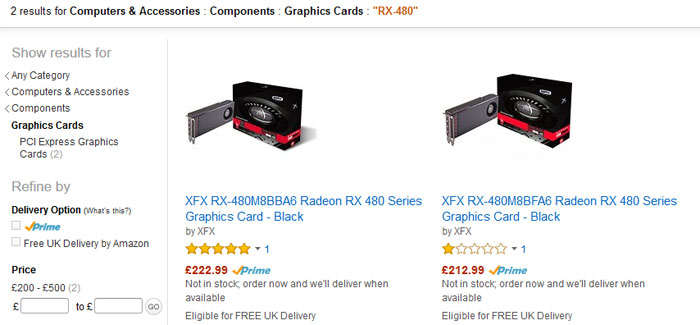The image depicts a webpage displaying search results for "Computers and Accessories, Components, Graphics Cards, RX-480." The results header is in black print, with "RX-480" highlighted in orange. On the left side of the page, there is a filter panel with various options: 

1. Categories, including "Computers and Accessories, Components, Graphics Cards."
2. Delivery options, specifically "Prime" and "Free UK Delivery by Amazon."
3. Price range options, allowing users to set minimum and maximum prices.

Further down, the webpage showcases two products side-by-side:

1. The first product is the "XFX-RX Radeon RX-480 Series Graphics Card, Black by XFX." It has a 5-star rating based on one user review and is priced at $22.99.
2. The second product is the "RFX-RX Radeon RX-480 Series Graphics Card by XFX," which has a 1-star rating based on one review and is priced at $212.99 with Prime delivery.

The page layout features a structured, easy-to-navigate format, aiding users in refining their search based on category, delivery options, and price.